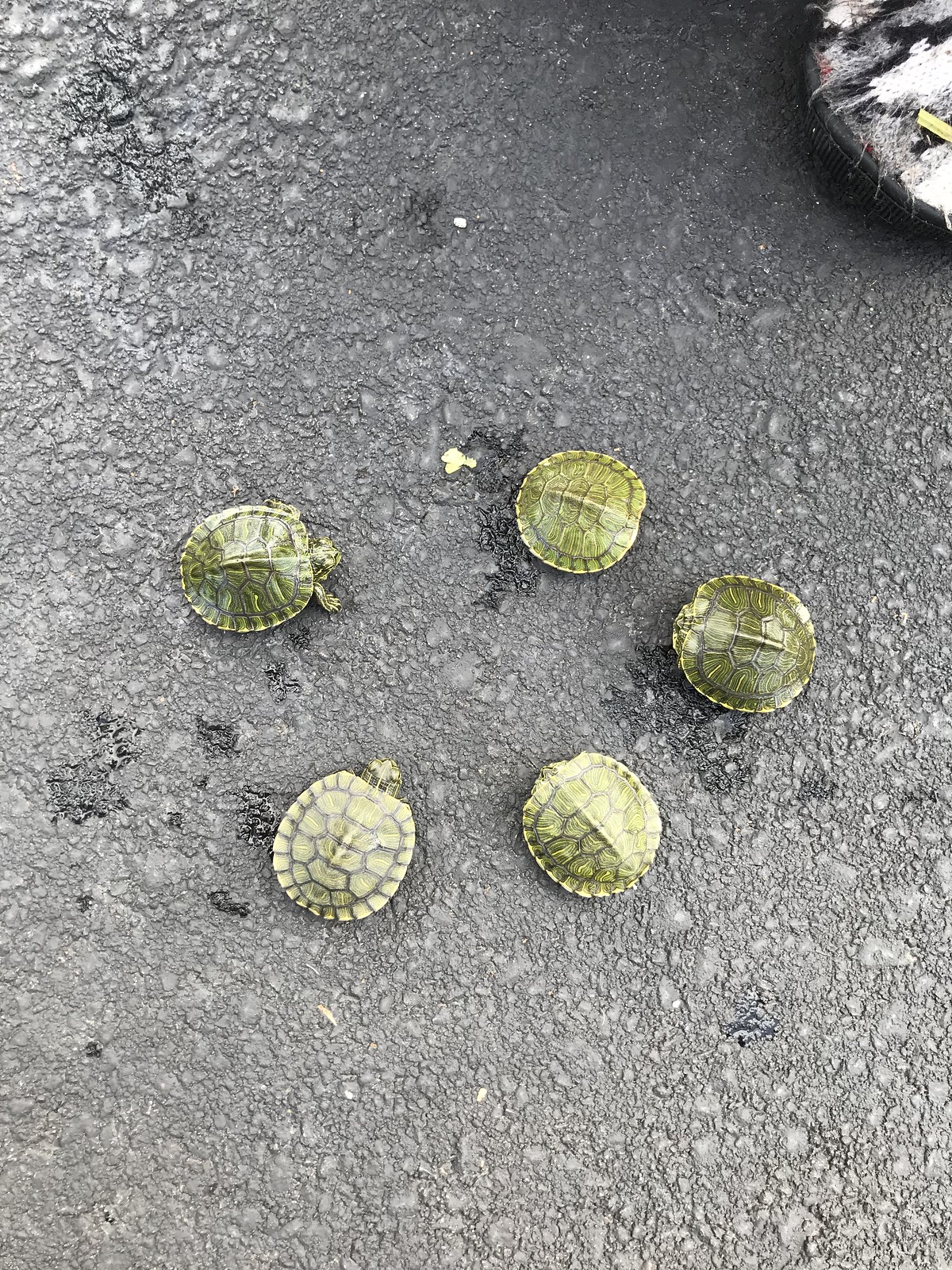This outdoor photograph captures five small turtles with green and patterned shells on a sunlit, dark gray pavement. The turtles are arranged in a loose circular formation. Two turtles have their heads poking out from their shells, while one has both its head and legs extended as if preparing to move towards another turtle. The remaining three turtles have retracted their heads into their shells. The shells exhibit intricate geometric patterns with darker spaces and lighter green areas, some featuring yellowish-golden spots. The pavement beneath them shows signs of wear with bumps and marks, and there appears to be an unidentified black and white container with some white substance in the upper right-hand corner. Bright sunlight bathes the scene, highlighting the turtles and their detailed shells against the worn pavement.